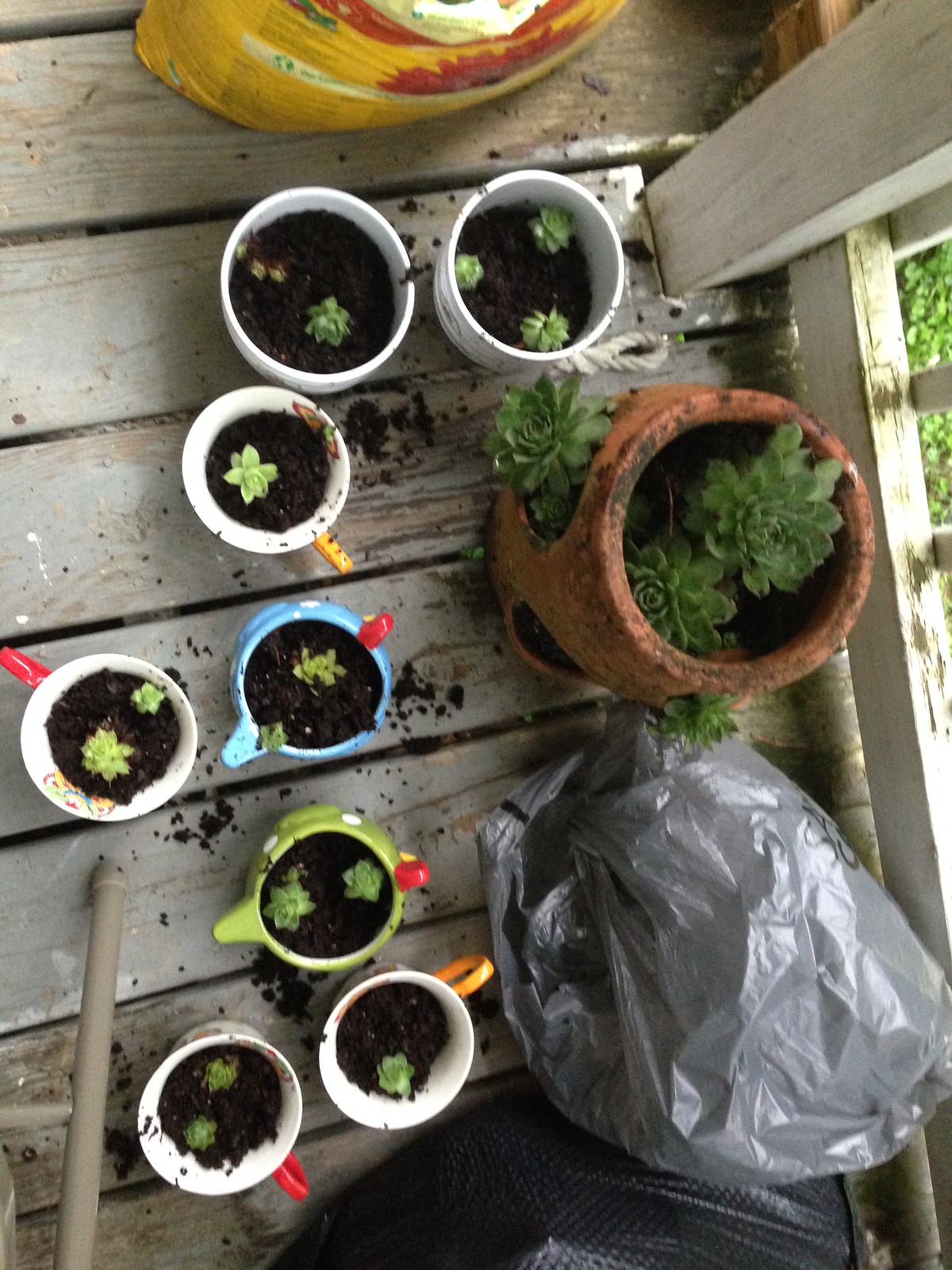The photo taken from an overhead perspective captures a semi-enclosed porch with weathered, graying wooden floorboards. On the right edge of the image, there's a white deck fence. The scene centers around various small planters that resemble mugs and teapots, each containing freshly potted succulents. Among these, there are six white pots, a light blue pot, a pale green pot, and a larger terracotta pot with side holes, typically used for strawberries. The planters feature handles in various colors—yellow, red, pink, orange, and green. Scattered soil and a plastic bag with gardening supplies suggest recent planting activity. A partially visible chair and some plastic-covered ladders frame the scene, completing the composition of this rustic gardening setup.